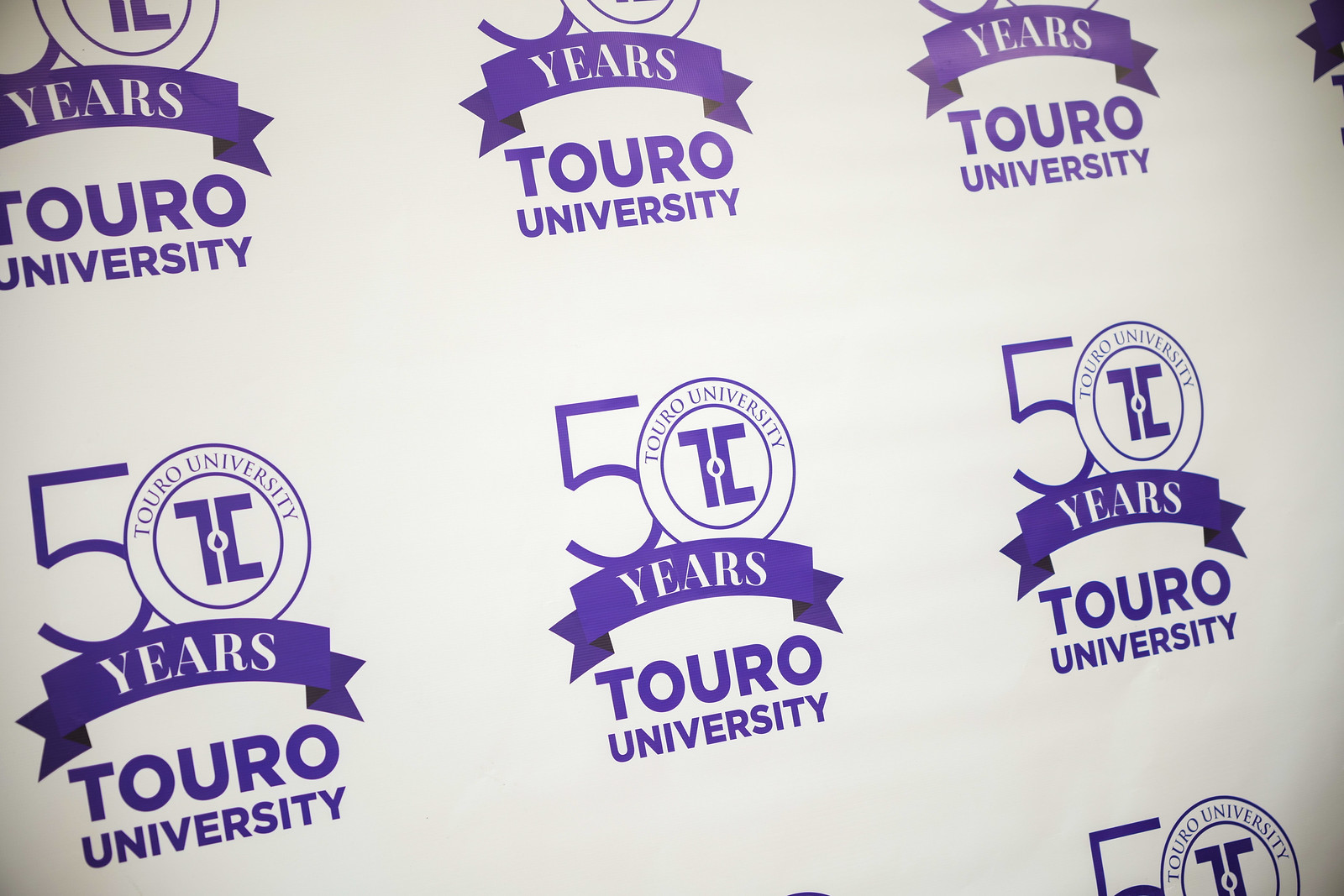The image features a detailed white backdrop patterned with a repeating purple logo commemorating the 50th anniversary of Touro University. Central to the design is the number "50" in prominent purple lettering, with the word "years" beneath it, also in purple. The "0" in "50" contains a distinct logo, which potentially represents Touro University, enclosed within two rings. Additionally, a purple ribbon runs across the composition, curving downwards, then upwards, and back down, adding a dynamic element to the design. The words "Touro University" (spelled T-O-U-R-O) are displayed in a serif font, wrapped around the top part of the "0" in "50". The background's minimalistic white and purple hues make the celebratory motif stand out, suggesting it might serve as a backdrop for events or photographs.